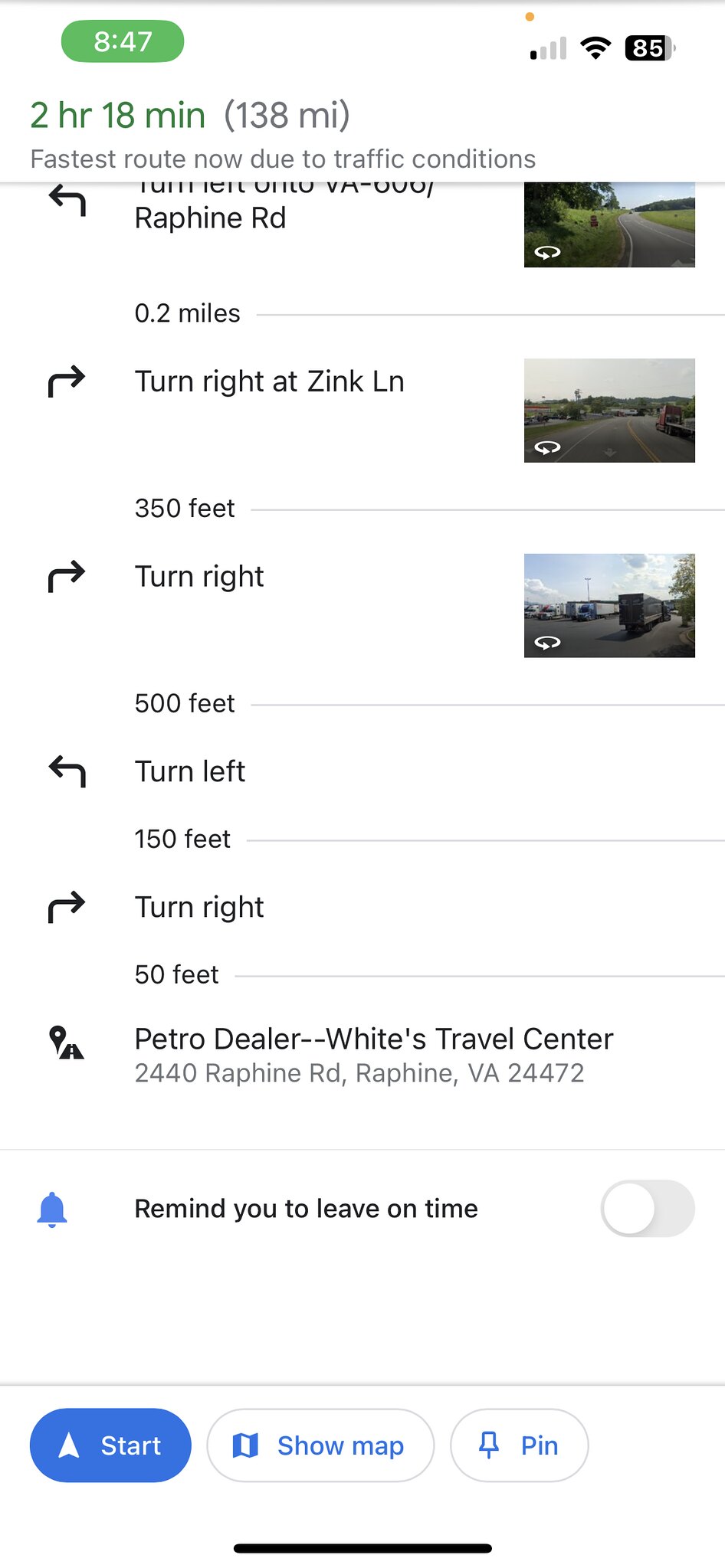This screenshot of a driving directions application on a phone displays detailed navigation instructions and various route information. At 8:47 AM, it indicates a 2-hour and 18-minute journey covering 138 miles on the fastest route due to current traffic conditions. The screen's top section, slightly cut off, includes a green banner with route details. The battery is at 85%, the Wi-Fi signal is full, and the cell signal shows one bar. Directions begin with a left turn onto Raffine Road, followed by multiple turns: right in 0.2 miles onto Zink Lane, right in 350 feet, left in 500 feet, right in 150 feet, and a final right turn in 50 feet leading to Petro Dealer White's Travel Center at 2440 Raffine Road, Raffine, Virginia, 24472. The page includes street-view images of rural two-lane roads bordered by grass and trees, a tractor trailer, and parking lot scenes with several parked tractor trailers. An option to set a reminder to leave on time is available, alongside buttons for "start," "show map," and "pin."